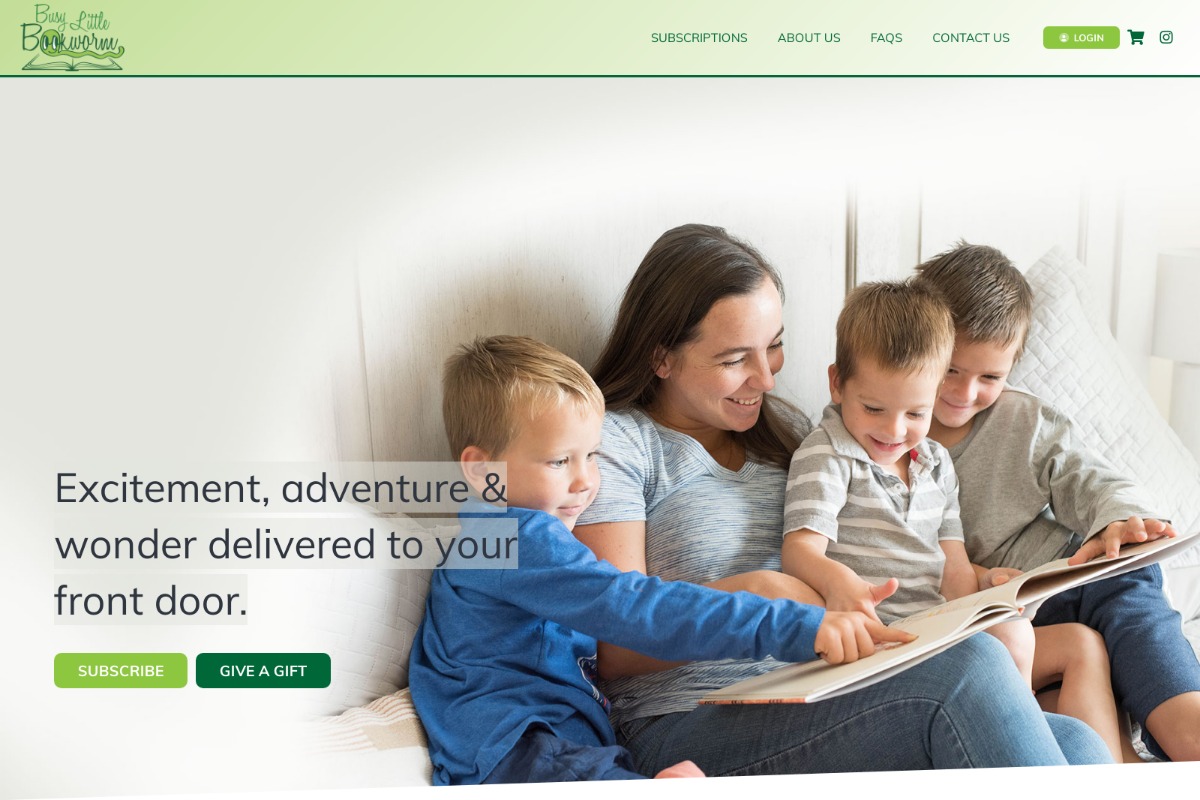This screenshot showcases the homepage of a website called "Busy Little Bookworm." The title is prominently displayed in green letters in the upper left corner, accompanied by a charming illustration of a worm with eyes perched atop a green book. On the upper right side of the page, there are menu options including "Subscriptions," "About Us," "FAQs," "Contact Us," and "Login." Additionally, there are icons for a shopping cart and Instagram.

At the center of the page, there is a heartwarming image featuring a woman who appears to be a mother, surrounded by her three young sons. They are all engaged in reading a book together, with the children either sitting on or very close to their mother. The boys are pointing at pictures in the book and smiling, while the mother also beams with joy. Behind them, three pillows and a lamp set an inviting and cozy atmosphere, suggesting they are comfortably seated on a bed, couch, or in a den.

On the left-hand side of the page, the text "Excitement, adventure, and wonder delivered to your front door" invites visitors to explore further. Below this message, there are options to "Subscribe" with a light green background and "Give a Gift" with a dark green background. Both options are written in white letters and emphasize the site's mission to deliver literary joy and familial bonding experiences directly to users' homes.